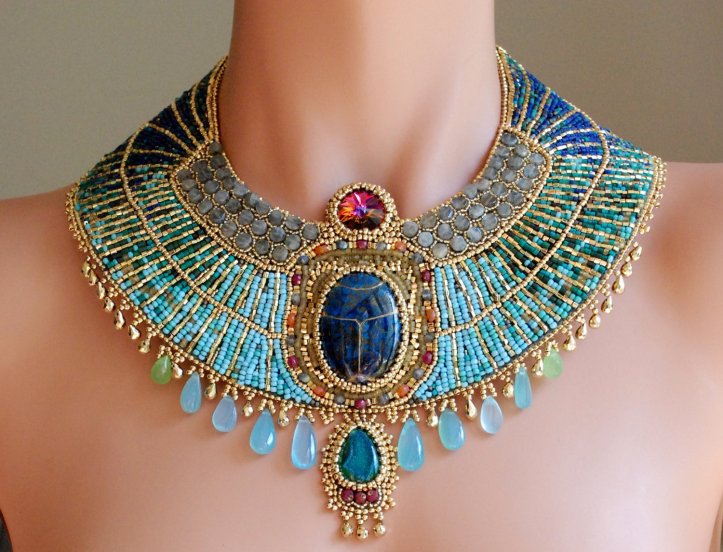The full-color photograph showcases an artistic close-up of a Caucasian woman's neck and shoulders, featuring a detailed and elaborate necklace. The background of the image is minimally gray on the upper right and left corners, making the necklace the central focus. The necklace is an intricate, Egyptian-themed piece adorned primarily with turquoise and sky-blue beads, giving it a multi-layered and textured appearance. At the top of the necklace is a striking red stone that appears to contain an explosion of colors, reminiscent of a rainbow. Beneath it is an oval-shaped, dark blue stone that resembles a scarab beetle shell, and further down is a smaller blue jewel. The necklace is thick and elaborately designed, with goldish beads accentuating the main stones. The bottom of the necklace features teardrop-shaped stones in various shades of blue, adding to its ornate and visually captivating design. Despite its intricate craftsmanship, the necklace is more pretty than valuable.